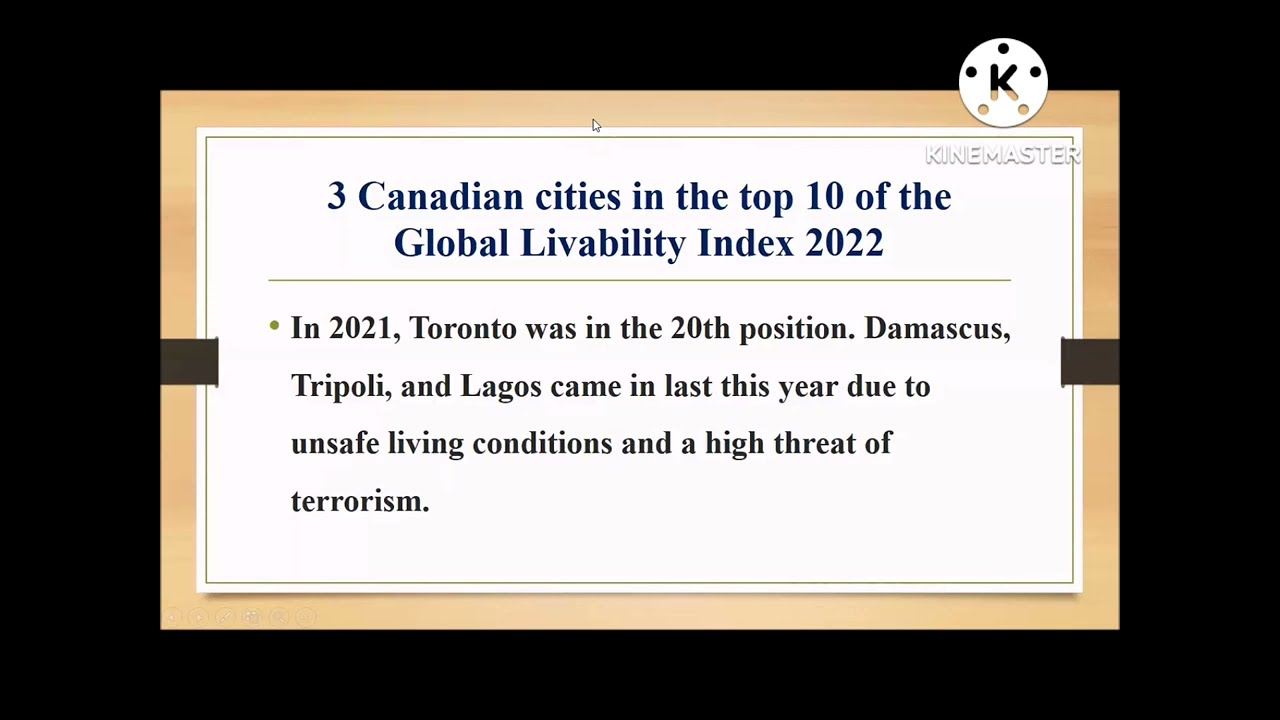This image is a screenshot from a video discussing Canadian cities' rankings in the Global Livability Index 2022. The background is entirely black, drawing one's attention to the significant elements of the image. In the upper right-hand corner, there is the logo for the video editing software "KineMaster," represented by a round white circle with five cut-outs along its circumference and a central cutout forming the letter "K." 

Beneath this logo, the words "KINE MASTER" are printed in white, clearly identifying the software used. Dominating the center of the screenshot is a horizontally placed rectangular section with a beige border and a white interior. Inside this section, black text delivers the crucial information: "Three Canadian cities in the top ten of the Global Livability Index 2022. In 2021, Toronto was in the 20th position. Damascus, Tripoli, and Lagos came in last this year due to unsafe living conditions and a high threat of terrorism." This comprehensive caption conveys both the triumph of Canadian cities in the Global Livability Index and highlights the contrast with cities that are struggling with severe safety and security issues.